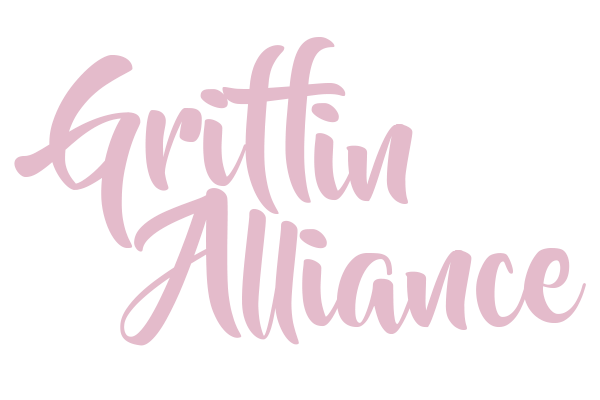The image features the words "Griffin Alliance" written in a quick, almost cursive style, reminiscent of neat, handwritten script. The text is centrally placed on a white, possibly transparent background. The letters are a dark pink or fuchsia color, creating a striking contrast against the white backdrop. The word "Alliance" is slightly indented, starting directly under the 'I' of "Griffin," giving a structured, professional appearance that suggests it might be a logo for a company.